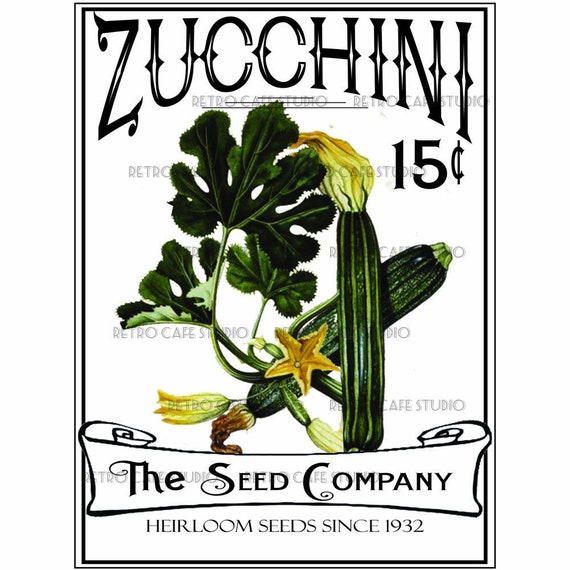This vertically rectangular advertisement features the word "ZUCCHINI" in large, stylized, black capital letters across the top, set against a plain white background. Below the title, to the right, the price "15 cents" is also displayed in black text. The center of the image showcases a collection of long, deep green zucchini, some with attached stems and yellow flowers, nestled among thick, dark green leaves. The bottom of the ad contains a banner with curled edges that reads "The Seed Company," followed by "Heirloom Seeds Since 1932" beneath it. Overlaying the entire image is a digital watermark that says "Retro Cafe Studio," indicative of a digital addition.